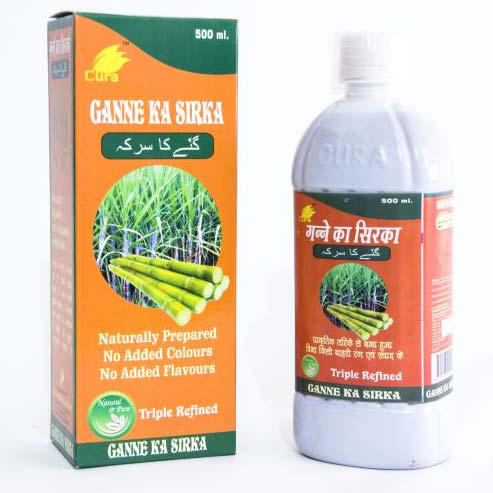The image features a natural herb product from India, prominently labeled as "Gane Ka Serka." The product appears to be a nutraceutical syrup, possibly derived from a plant that resembles asparagus or bamboo shoots, although its actual botanical source might be different. The packaging consists of a large, orange box with green accents on the top and bottom, displaying the product's name in both English and another language. The box highlights key features: "naturally prepared, no added colors, no added flavors, triple refined." The bottle, positioned to the right of the box, mirrors the same design elements and text. The bottle itself is white plastic with a green and orange label, consistent with the design on the box, and has a white cap. The box also mentions the volume, indicating that it contains 500 milliliters of the product. Overall, the image depicts an intricately designed, well-labeled herbal supplement product that emphasizes its natural preparation and purity.